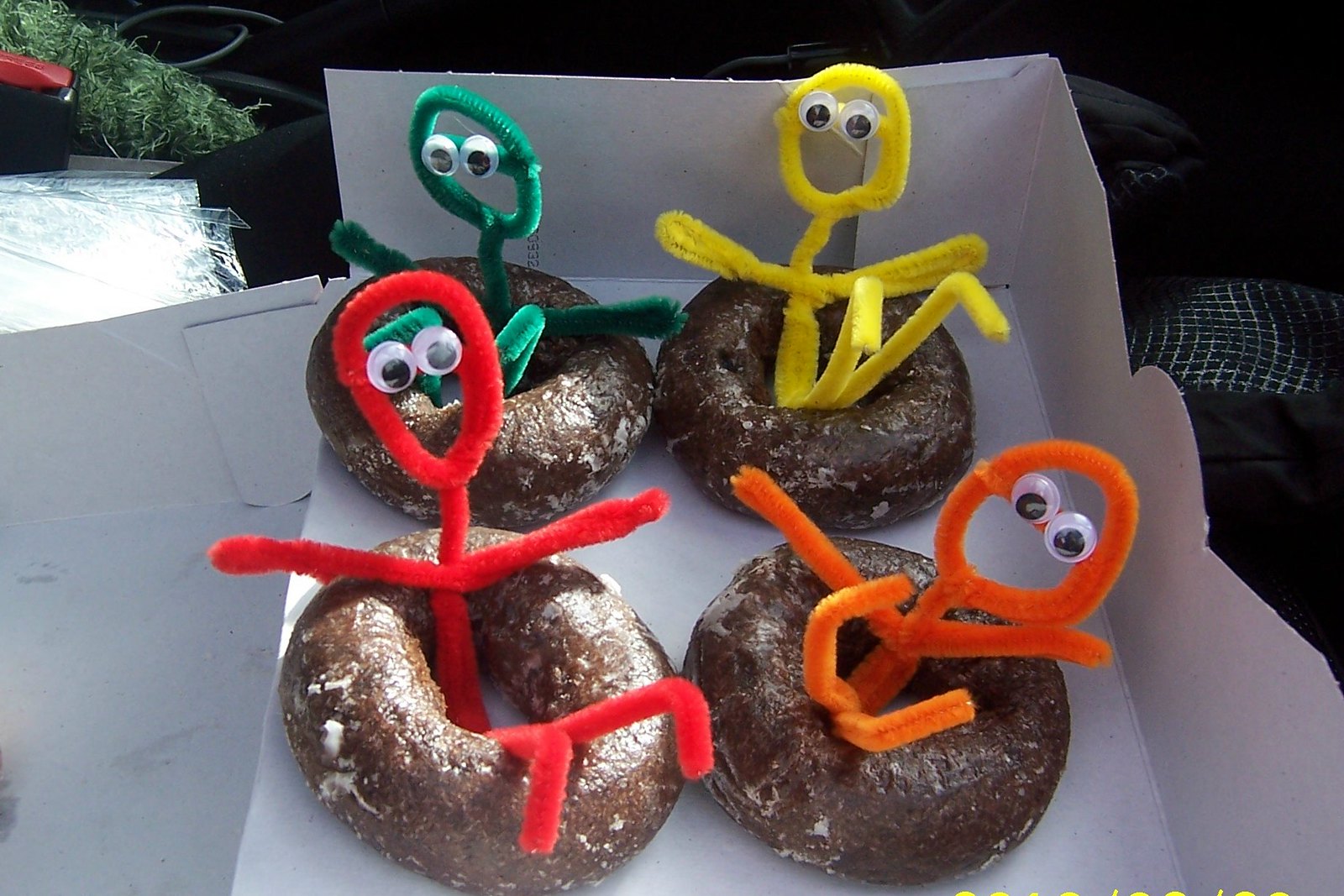The photograph depicts a white cardboard bakery box sitting on a table in an outdoor setting, with subtle background details including some leafy greenery and indistinct plastic and dark objects. Inside the box, which is ripped open, are four glazed chocolate cake doughnuts, each featuring a colorful stick figure made from pipe cleaners – red, orange, yellow, and green. Each stick figure, complete with googly eyes, is positioned as if tubing within the ring of its respective doughnut, giving a whimsical and playful touch to the scene. The simplistic yet intriguing setup of the photo emphasizes the contrast between the detailed doughnut decorations and the plain outdoor backdrop.